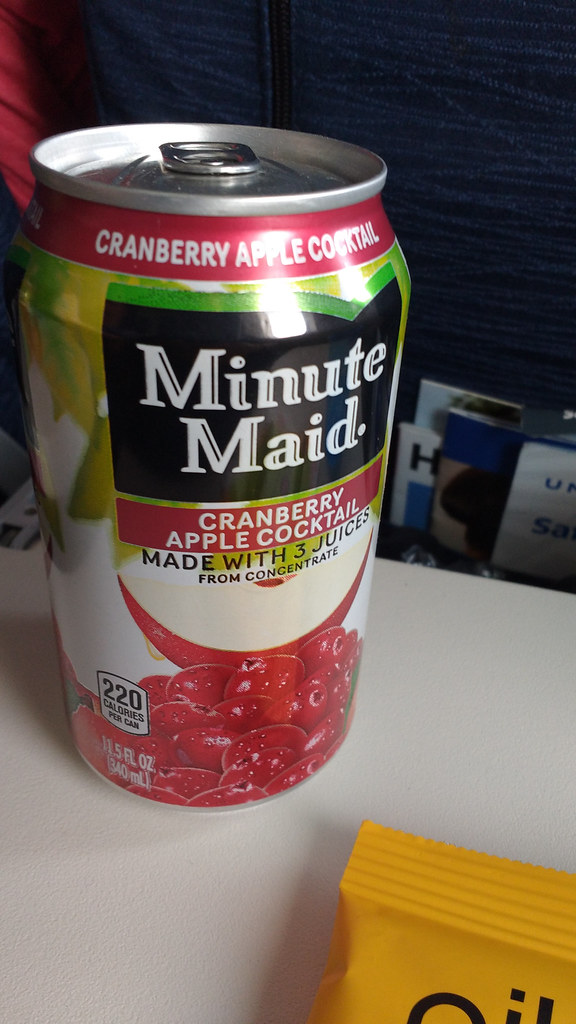This is a vertically oriented, rectangular photograph prominently featuring a can of Minute Maid Cranberry Apple Cocktail. The can is placed centrally within the frame, standing on a white countertop. Its design prominently displays a cluster of cranberries at the bottom, accompanied by a label indicating that the drink contains 220 calories per can. The can has a capacity of 11.5 fluid ounces or 340 milliliters. Moving upwards from the imagery of cranberries, there is text stating "Made with 3 Juices From Concentrate," followed by the product name, "Cranberry Apple Cocktail." The Minute Maid logo is clearly visible below this text. Encircling the top rim of the can is a red band with white lettering that repeats the product name, "Cranberry Apple Cocktail." In the bottom right-hand corner of the image, an orange package with black writing is partially visible, though its purpose or contents remain unclear.